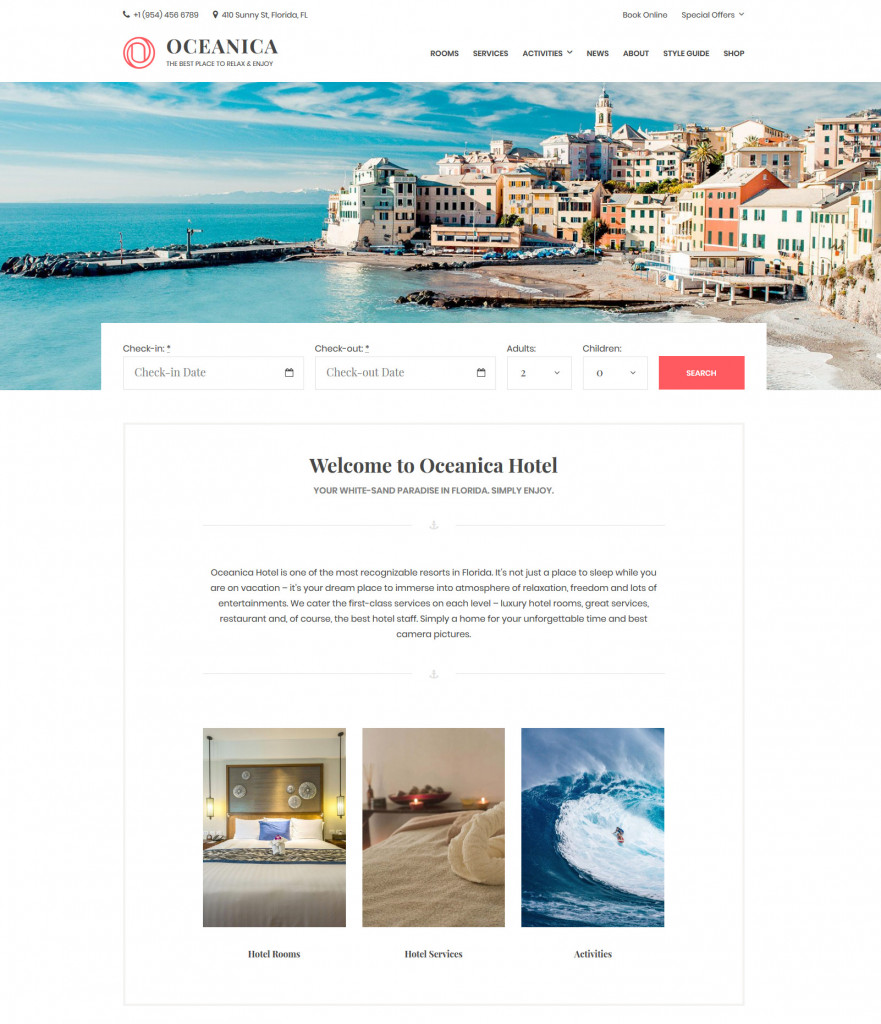**Website Caption for Oceanica Hotel:**

At the top of the computer screen, a white banner stands prominently displaying the hotel’s essential contact information alongside the title "Oceanica: The Best Place to Relax and Enjoy," all written in sleek black text. Above this are navigational links in black, offering pathways to sections such as Room Services, Activities, News, About, Style Guide, and Shop. To the right, buttons for "Book Online" and "Special Offers" are easily accessible.

The main visual attraction is a stunning picture of a seacoast bathed in turquoise water under a radiant blue sky adorned with pastel clouds. The landscape transitions from sands of coral and white to buildings of varied heights, rooflines, and window sizes, each facade contributing to a charming and diverse coastal scene. Docks and what appear to be dune buggies are visible in the foreground. The picturesque setting includes a rocky coast and a jetty extending into the glistening water, with the sun casting a glimmering trail on the waves and a hint of a sandy beach in view.

Below this captivating image, a user-friendly booking interface displays tabs for entering check-in and check-out dates, as well as the number of adults and children, complemented by an orange search button. Beneath this, a welcoming message reads: "Welcome to Oceanica Hotel, your white sand paradise in Florida."

The accompanying text enriches the experience, describing Oceanica as one of Florida’s most recognizable resorts, where visitors can immerse themselves in an atmosphere of relaxation, freedom, and entertainment. The statement highlights the hotel's first-class services across all levels, luxurious rooms, superb dining, and the best hotel staff, aiming to make every moment unforgettable and perfectly captured.

Following the description are three inviting images: the first shows a large bed adorned with two white pillows and one blue pillow, complemented by art above the headboard and a hanging lamp to the left. The second image features candles on a dresser and a meticulously arranged bedspread. The third image depicts someone surfing a massive wave. Below these images, links to Hotel Rooms, Hotel Services, and Activities are clearly displayed.